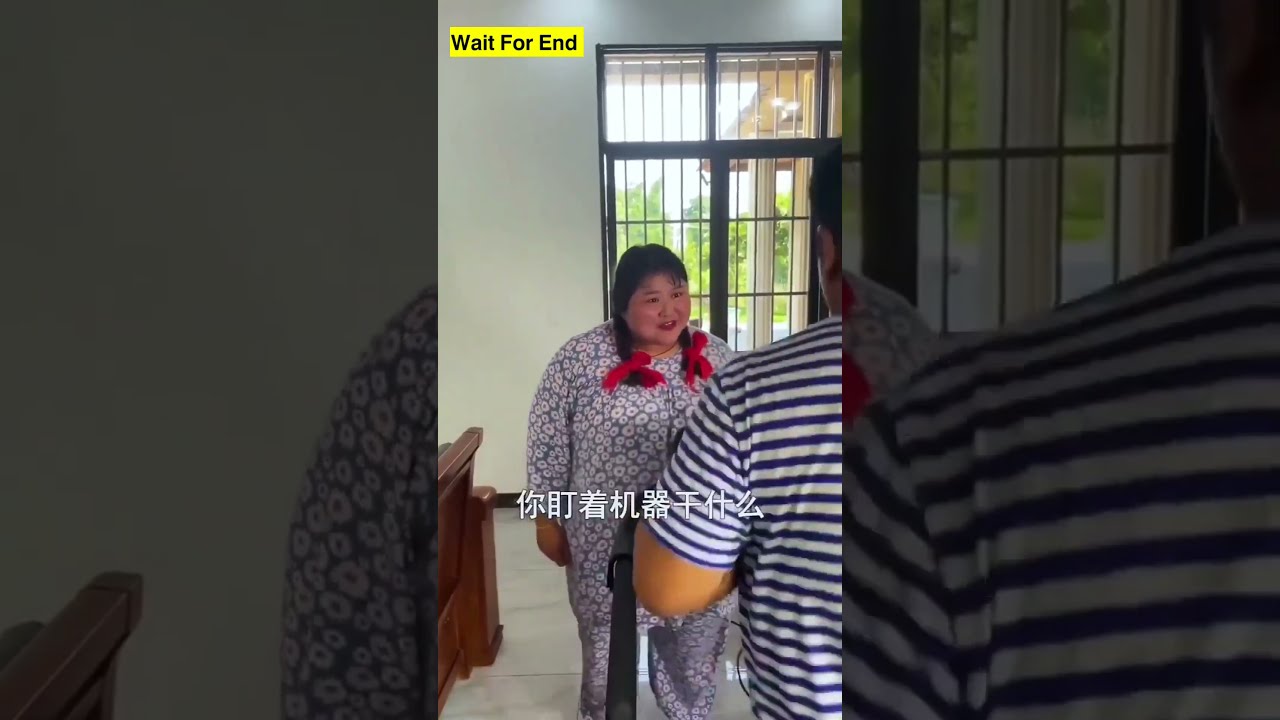In the screenshot from what seems to be an Asian drama, there is an Asian woman wearing long-sleeved, floral-patterned gray pajamas with red ribbons tied around her two braids. She appears to be heavyset and is facing a man whose back is to the camera. The man, who has short hair, is dressed in a blue and white striped t-shirt, and you can only see his left arm, a part of his left ear, and a glimpse of his neck. Behind the woman is a large black-framed window or doorway through which grass and pillars are visible. The setting looks somewhat formal, potentially a church or courthouse, given the presence of a blue wooden pew and a mahogany bench seat. The floor is gray, and a wooden stand is nearby. The image is overlaid with the text "wait for end" and features some Asian characters, potentially Japanese or Chinese, in the center. The colors in the scene include white, blue, black, green, skin tones, brown, and gray.